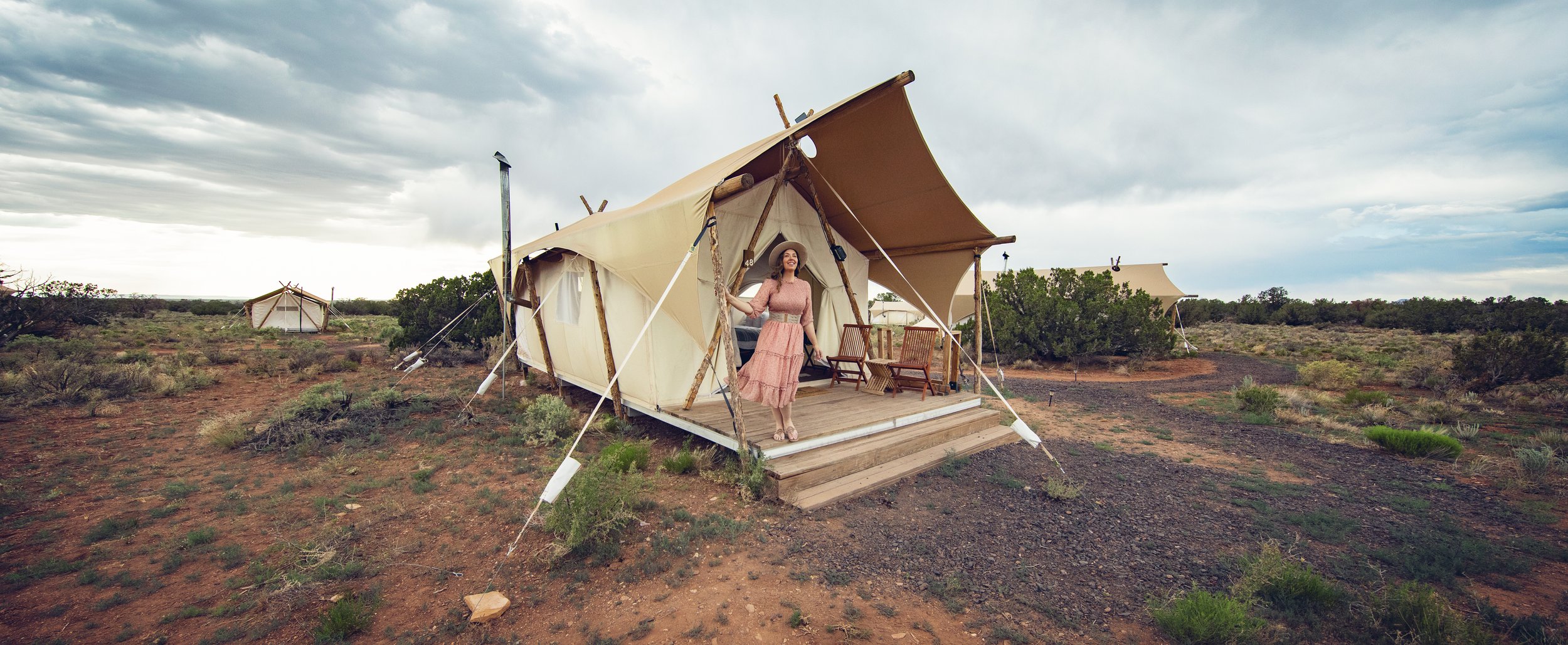The panoramic photograph captures a modest dwelling or trailer home set in a remote, arid landscape, surrounded by dirt, rocks, and sparse scrub vegetation. The central focus is a woman in a pale pink dress with a straw hat, standing on a small porch. She holds onto the edge of the porch, seemingly taking in her surroundings. The porch is furnished with a couple of wooden chairs. The dwelling is covered by a canvas awning secured with ropes to provide shade. The awning, resembling a large tent, is supported by numerous lines staked into the ground. The dwelling also features a small pipe, likely connected to a wood stove. In the background, there are green bushes and a mix of cloudy and blue skies, suggesting an overcast day. Additional small structures are visible to the left, including a white one with a brown roof and another structure with a tan roof beyond some trees. The overall scene suggests a peaceful, quiet moment amidst vast, open space devoid of modern amenities.